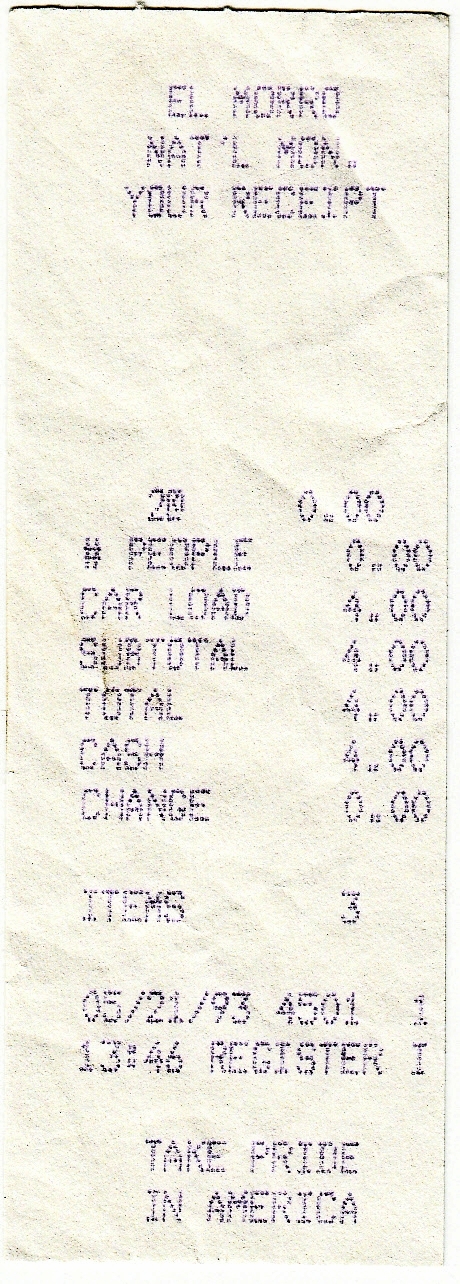This is a detailed image of a slender, old paper receipt from El Morro National Monument, printed in blocky blue ink. The receipt, which appears to have been folded several times and sports a small stain near the subtotal, has a vertical rectangular layout with a white background. At the top, it reads "El Morro National Mon." (short for monument) followed by "Your Receipt." It lists a few items: 

- Number of people: 0
- Car load: $4.00
- Subtotal: $4.00
- Total: $4.00
- Cash: $4.00
- Change: $0.00
- Number of items: 3

The receipt is dated "05/21/93" at "13:46" (military time) from register one. At the very bottom, it carries the patriotic slogan, "Take Pride in America."